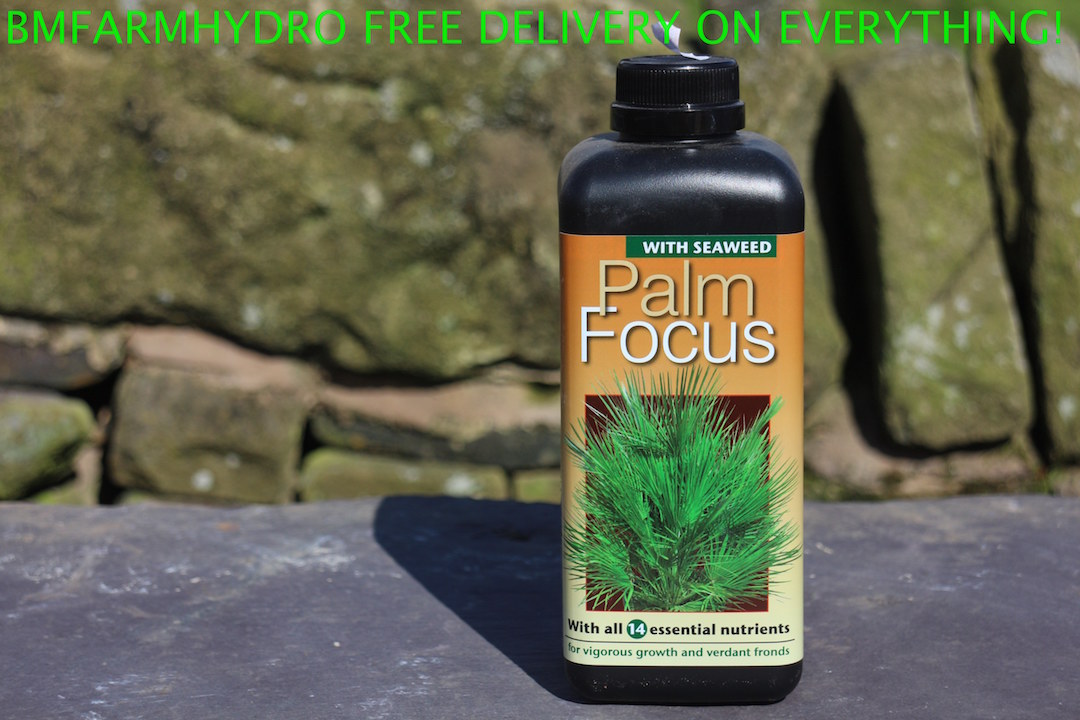In the center of the photograph stands a black, rectangular bottle prominently featuring an orange label. The label transitions to a lighter gradient towards the bottom, where it displays a green palm tree amidst an image of verdant fronds. The label text describes the product as containing seaweed and palm focus, and boasts "with all 14 essential nutrients for vigorous growth and verdant fronds." Above this central image, the label bears a green inscription reading "BMF Farm Hydro - Free delivery on everything!" The bottle is positioned on a table with a black surface, set against a backdrop that includes a natural setting of intricately stacked rocks, resembling a rock wall. This earthy background complements the natural theme of the product, likely plant food, designed to nurture plant growth.